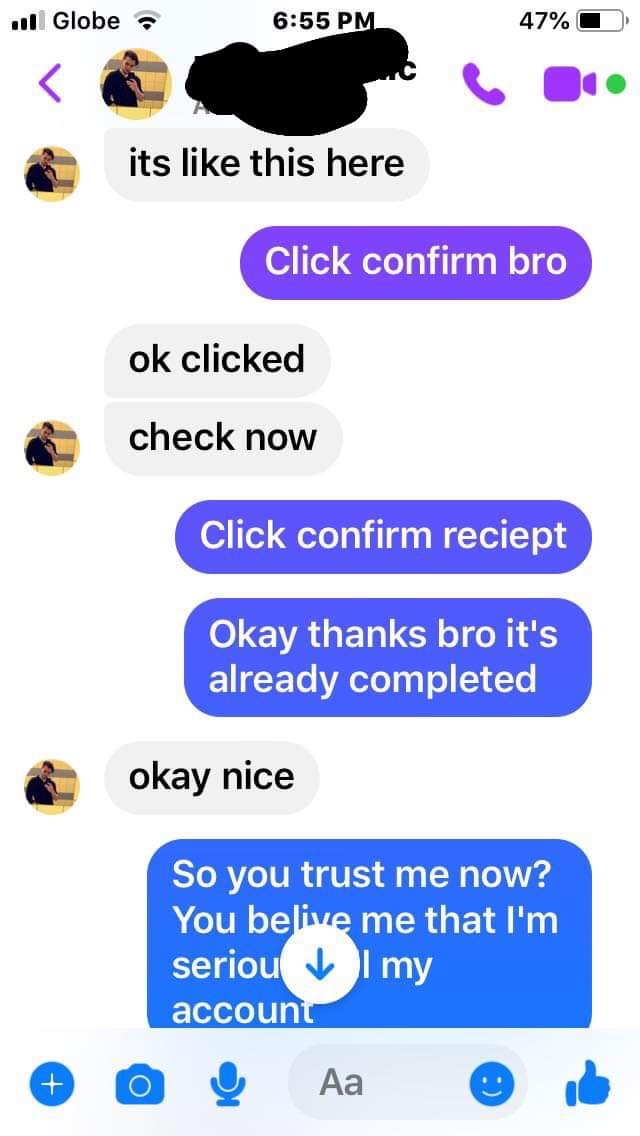A detailed screenshot of a Facebook Messenger conversation on an iPhone, displaying a messaging interface with two individuals chatting. At the top of the screen, it shows the carrier as Globe, the time as 6:55 PM, and the battery at 47%. The conversation involves instructions to confirm an action. One participant repeatedly asks the other to "click confirm, bro," "check now," and "click confirm receipt," to which the other replies with confirmations and gratitude, saying, "Okay, clicked," and "Thanks, bro, it’s already completed." Different messaging features are visible at the bottom, including icons for a camera, a plus sign inside a circle, 'AA' text options, and a blue smiley face. The background is white, highlighting the text bubbles in blue and purple. The conversation ends with a query about trust and account verification.